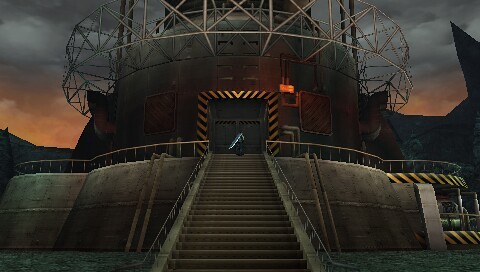The image features a rounded building positioned centrally in the background. Surrounding the building is a metal gate with bars arranged in an X pattern. A prominent black door, bordered by yellow and black caution stripes, serves as the building's entrance. A staircase, accompanied by silver-colored handrails, extends from the bottom center of the image, leading up to the door. Handrails also line the exterior of the building. The sky above displays a blend of gray and orange hues, adding a moody atmosphere to the scene. Additional yellow and black caution stripes are visible on the right side of the image, enhancing the industrial feel.